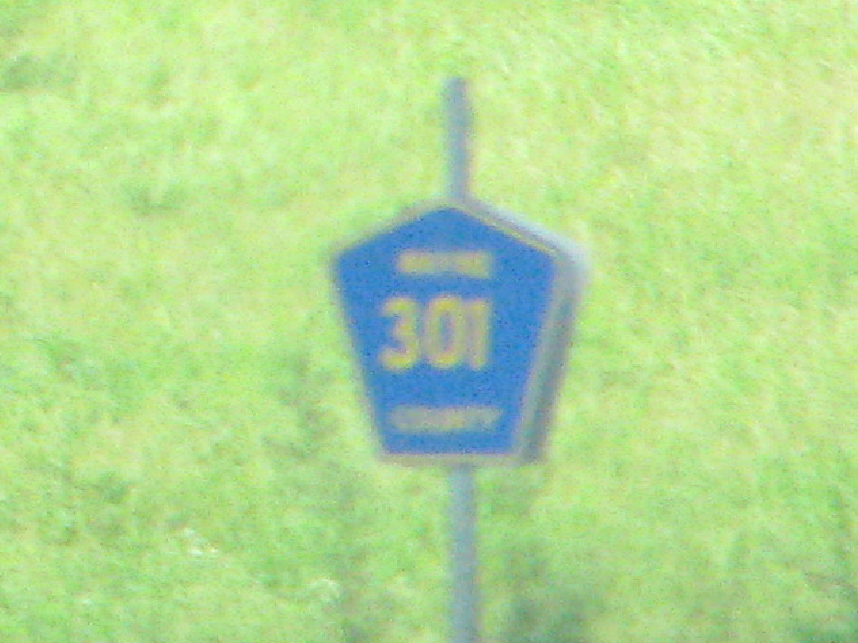The photograph depicts a blurry and hazy image of a unique five-sided highway sign, mounted on a silver cylindrical steel post. The sign features a blue background with yellow print, displaying the number "301" prominently, followed by the word "County" underneath. Above the number 301, a word appears that could be the name of the county, but it is illegible due to the image's poor quality. The background reveals a grassy field bathed in bright sunlight, with grass appearing light green to almost yellow. The field may suggest the photo was taken from a moving vehicle, contributing to the blurriness.